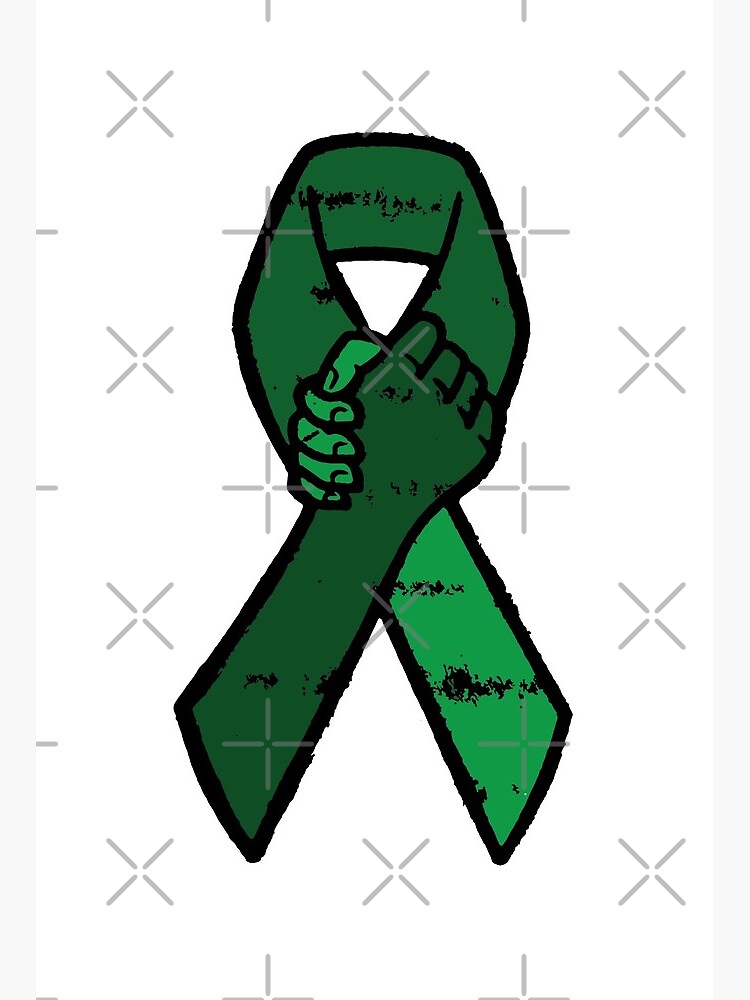This is a digital mock-up or prototype image of a green ribbon, heavily stylized to represent unity and solidarity. The ribbon, reminiscent of an AIDS or breast cancer awareness ribbon, features a dark green hand and a lighter green hand clasping together where the ribbon would traditionally overlap, forming a combined fist. The ribbon itself is outlined with a thick black line, and the fabric of the ribbon is adorned with distressed black stylized lines, adding texture and depth. The background is completely white, and a semi-transparent watermark of gray crosses and X's is repeatedly overlaid on the image, likely to prevent unauthorized usage. The overall appearance suggests that this digital artwork was created in Illustrator and may serve as a printing proof or prototype.